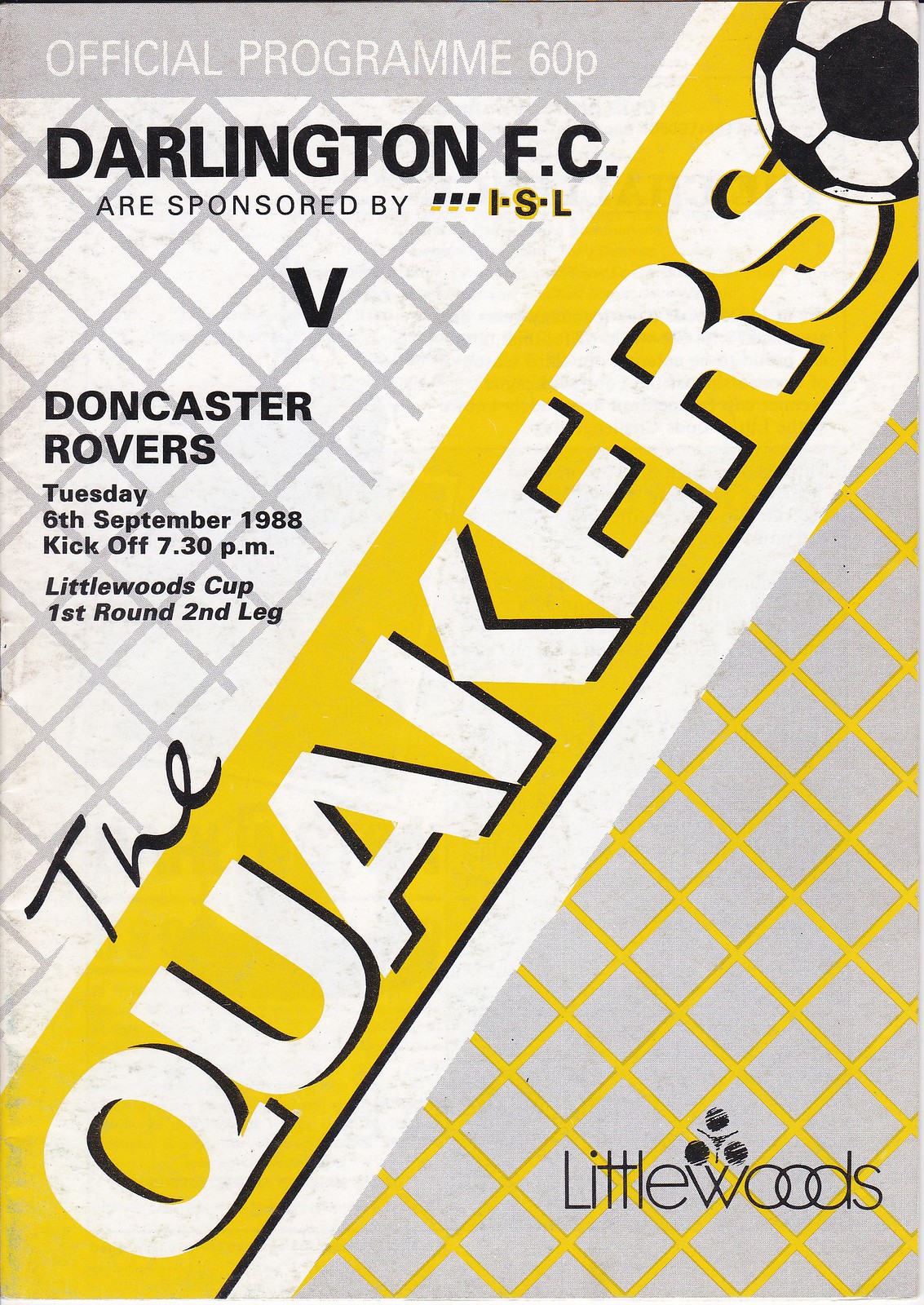Here is a detailed and cleaned-up single caption for the image:

The image is a scan of a poster, likely for a football (soccer) match. It is vertically oriented with a gray background, designed to resemble a soccer net. At the top, in white text on a gray banner, it reads "Official Programme" (notably spelled with an extra 'mme'), priced at 60 pence (60P), indicating a British origin. Below this, in black text, it states "Darlington FC are sponsored by ISL" followed by "V" (versus) "Doncaster Rovers." The match details include "Tuesday, 6th September 1988, kickoff 7.30 PM, Littlewoods Cup, first round, second leg." A prominent yellow diagonal banner stretches from the lower left to the upper right corner, with the word "The Quakers" in white text and a soccer ball beside the 'S'. In the lower right, the text "Littlewoods" appears on a gray background with diagonal yellow Xs, and a logo featuring three dots with lines separating them. This program could have been purchased for the 1988 football match between Darlington FC and Doncaster Rovers.